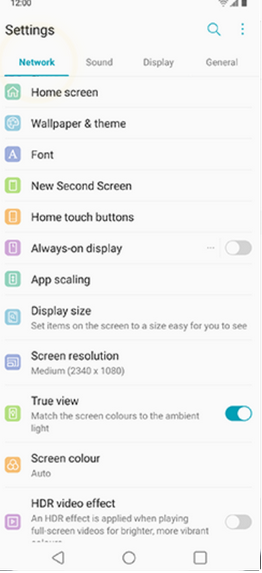The image depicts a settings screen of a device, displaying various configuration options. At the top of the screen, status indicators show the current time, Wi-Fi connectivity, and the word "Settings" in black text. Adjacent to the title, a blue magnifying glass signifies the search function, and three vertical blue dots represent more options.

The main section of the screen is divided into different settings categories, with "Network" highlighted in blue, suggesting it to be the currently selected option. Below the primary settings categories, there are multiple configurable elements each accompanied by distinct icons:

1. **Home Screen**:
   - Icon: Green background with a white house.

2. **Wallpaper and Theme**:
   - Icon: Blue, resembling a circle.

3. **Font**:
   - Icon: Purple background with a white "A".

4. **New Second Screen**:
   - Icon: Lime green.

5. **Home Touch Buttons**:
   - Icon: Orange with a smartphone on it.

6. **Always On Display**:
   - Icon: Pink with a smartphone, with the function turned off.

7. **App Scaling**:
   - Icon: Green.

8. **Display Size**:
   - Description: Adjusts items on screen for better visibility, with a blue icon.

9. **Screen Resolution**:
   - Description: Sets the resolution to Medium 2340x1080, with a purple icon.

10. **True View**:
    - Description: Matches screen colors to ambient light, with this setting turned on.

11. **Screen Color**:
    - Description: Set to 'Auto', with an orange icon containing three white circles.

12. **HDR Video Effect**:
    - Description: Enhances full-screen videos for brighter, more vibrant visuals, currently turned off, with a purple icon.

At the very bottom of the screen, navigation controls are displayed in gray: a back arrow, a circle, and a square.